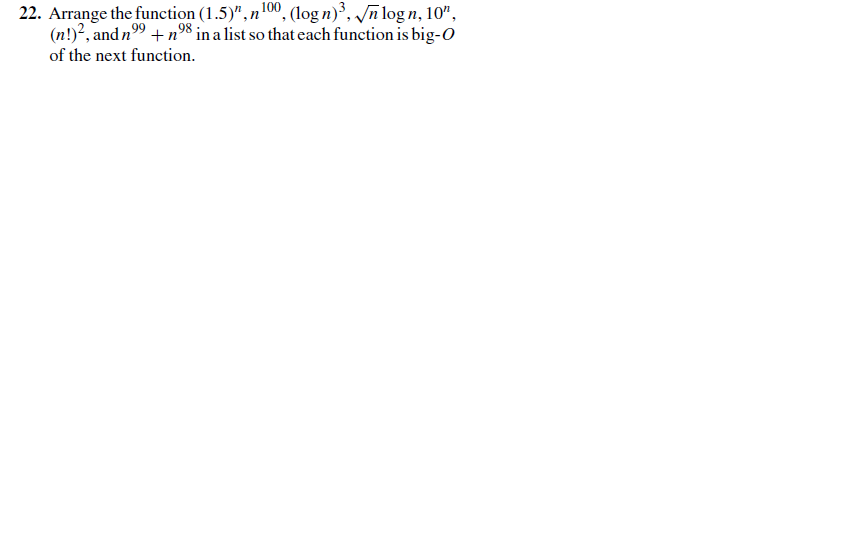The image is set against a plain white backdrop and features prominently, in the upper left-hand corner, black textual content presenting a mathematical problem. The initial part of the text reads '22.' in bold black font, signaling the start of a listed item. Following this, in a slightly less bold but still black font, is the main body of the text. It instructs to "Arrange the function (1.5)^n, n^100, (log n)^3, √n, log n next to √n but not underneath, 10^n, (n!)^2, and n^99 + n^98 in a list so that each function is a Big O of the next function." This list appears to be intended to order the growth rates of various functions with respect to complexity.